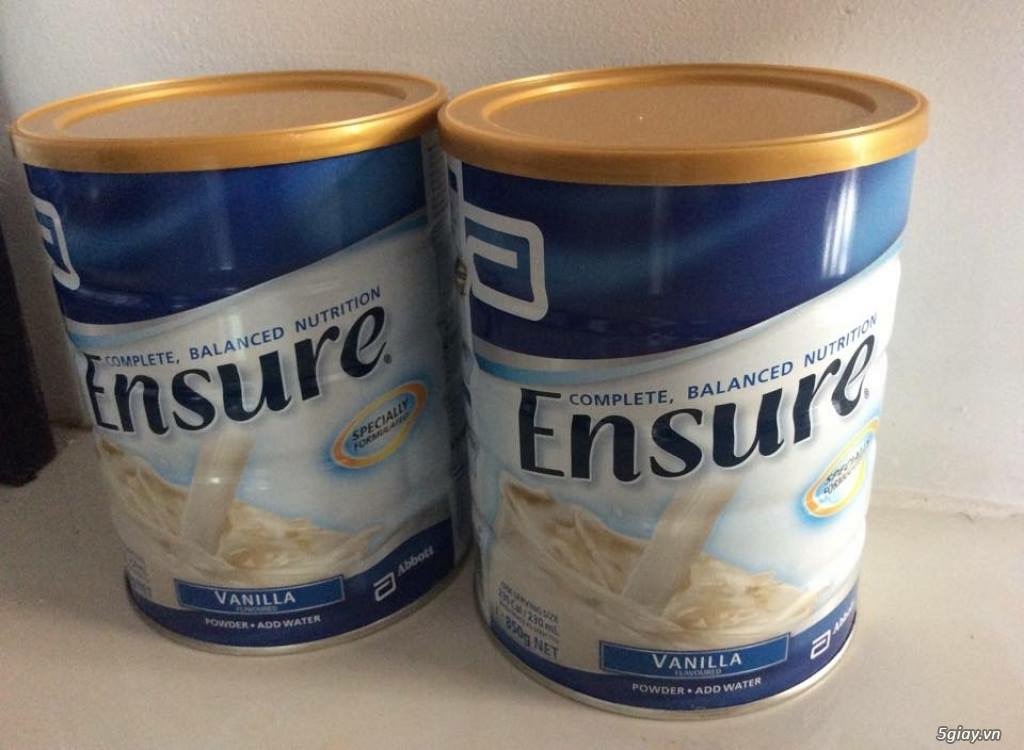The image depicts two identical canisters of Ensure, a nutritional drink, positioned on an off-white or beige surface with a white or light gray wall in the background. The canisters feature gold plastic lids that snap into place and labels that are predominantly blue and white with touches of yellow. The labels prominently display the words "Complete Balanced Nutrition" in blue letters and "Ensure" in bold black letters. Near the bottom of the labels, within a blue box, the word "Vanilla" is written in white letters, followed by instructions that read "Powder, add water." Each canister also has an image of a white liquid being poured into a similar milky liquid, indicating the drink’s preparation. The canister on the left is angled slightly towards the left, and the one on the right is angled slightly towards the right. In the bottom right corner of the image, there is text reading "5GIAY.VN." Additionally, a small black edge of an unidentifiable object is visible next to the left canister.